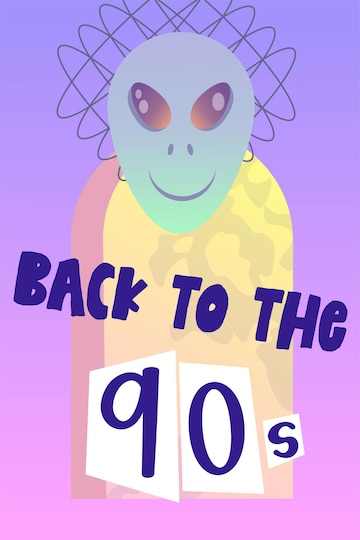The image is a computer-generated graphic featuring a vivid, gradient background that transitions from purple at the top to a lighter purplish-pink towards the bottom. Dominating the scene is an alien figure with a green head characterized by large, oval, slanted eyes, two small nostril dots, and a thin black smile. Swirly lines animate the space behind its head. The alien's body is depicted with a yellow semi-circle at the top that forms shoulders, and has a flat bottom. Over the chest area of the body, in dark purple, angled uppercase letters, it reads "BACK TO THE" followed by "90S" written within three white asymmetrical squares. There is a subtle, grayish pattern within the yellow part of the body, adding some texture to the otherwise simple design.